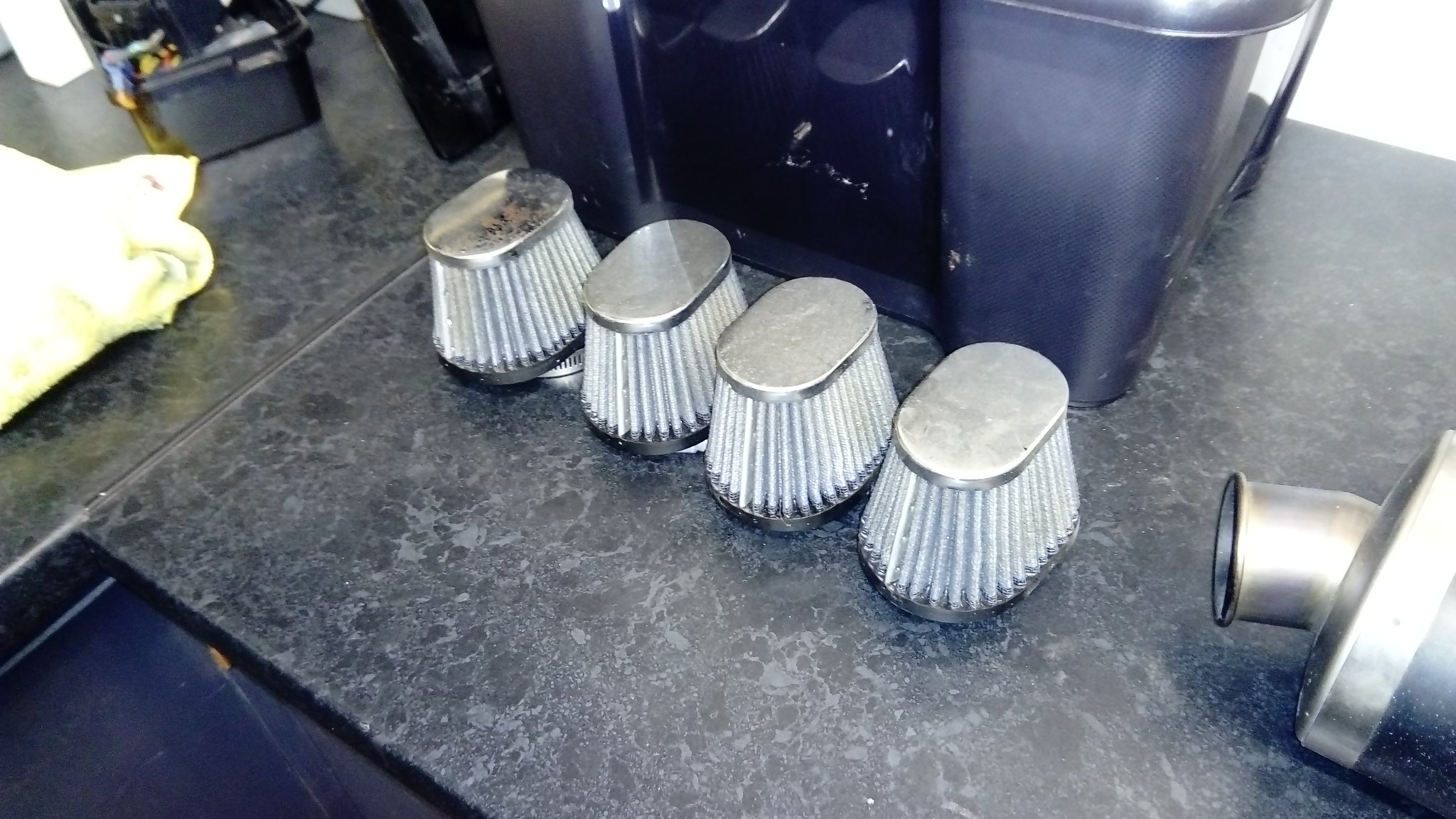The image depicts a close-up of a grey, dark grey marble-effect kitchen countertop. Central to the composition are four upturned, silver ridged metal objects that may resemble filters or perhaps cake casings. These are neatly arranged in front of a stainless steel, round machine, the exact nature of which is not easily discernible. In the background, there is what looks like a dark blue countertop water filter with several components. To the right of the setup is a black bucket containing what appears to be cleaning supplies, while to the left, a yellow cleaning rag or dish towel can be seen. The lighting in the room is on, casting clarity on the items, but leaving some details still ambiguous.